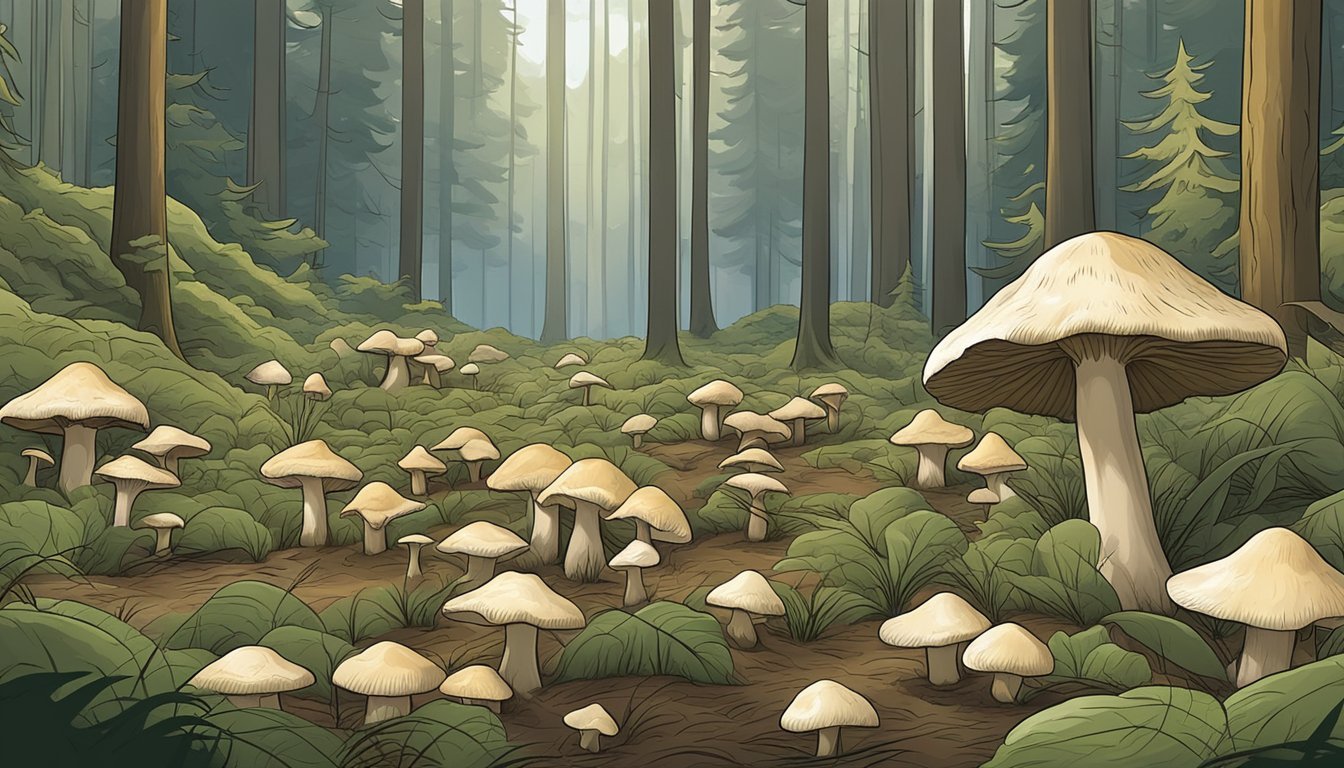This digital artwork depicts a serene forest scene bathed in muted, dim lighting. The foreground is lush with an understory of green plants with large leaves, their vibrancy subdued by the overcast ambiance. Intermixed among the verdant undergrowth, a variety of mushrooms pepper the forest floor, ranging from small to medium to notably large specimens. These mushrooms are predominantly a light beige and white color. Stretching into the background are the tall trunks of old-growth pine trees, their heights extending beyond the frame and hinting at the forest's grandeur. Also visible are shorter evergreen trees interspersed among the pines. To the left, a slight elevation in the terrain suggests a hilly area cloaked in grass and fallen leaves. The soft brown dirt beneath the foliage blends seamlessly with the scene, completing this tranquil, nature-filled illustration.